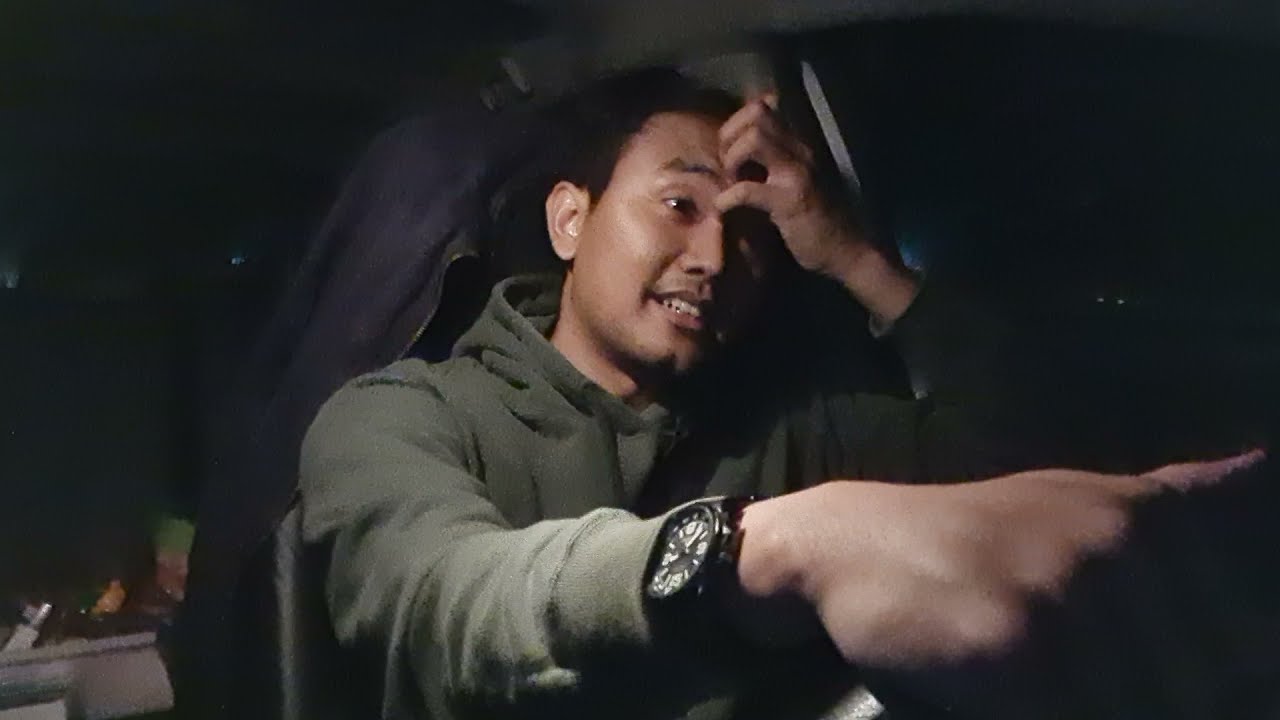The image depicts an Asian man in a close-up view, dressed in a greenish hoodie with a high collar and long sleeves. He has very short dark hair, bushy eyebrows, and appears to be seated in a gray seat, possibly within a car at nighttime due to the dark surroundings. The man’s facial expression shows a mixture of concern and intensity, as he might be clenching his jaw or smiling anxiously. His left hand, with fingers in a scratching motion using his middle, ring, and pinky fingers, touches his face, while his right hand, closer to the foreground, appears to be grabbing or pointing at something. This right hand also wears a black analog watch. The left side of his face is more illuminated, while the right side is shadowed. In the background, to the bottom left corner, there is a white drawer or desk with various items including a white bottle, and a brown basket containing orange and green objects. Behind him, a black jacket appears to be falling down.